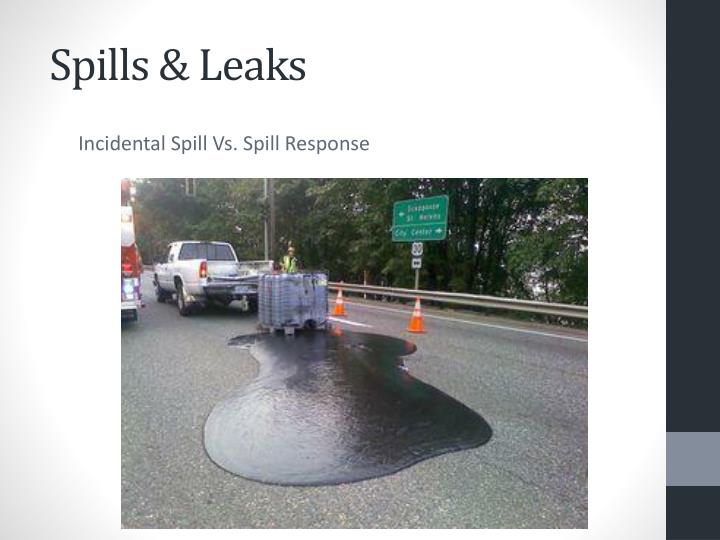The image, titled "Spills and Leaks", depicts an oil spill incident on a highway. Dominating the upper left corner of the rectangular photograph, dark gray or black text reads "Spills and Leaks," with the subtitle "Incidental Spill versus Spill Response" right below it in lighter gray lettering. To the right, a border of dark navy blue, almost black, with a gray strip at the bottom, frames the scene.

In the picture, the back of a silver pickup truck is prominently visible. Next to it is a container from which a thick, dark tar-like oil has spilled onto the asphalt, creating a puddle. In the foreground, a man equipped with a green fluorescent vest and a hard hat stands near the spill, seemingly assessing the situation. There are two orange traffic cones placed on the right side of the spill, close to a safety rail that extends along the highway. Above the safety rail, a green interstate sign can be seen. 

In the backdrop, at the center, there is a street sign indicating US-30, visible amidst the trees. The highway scene is set against a light gray background, enhancing the visibility of every detail and emphasizing the severity of the spill. The overall ambiance suggests an emergency response underway during daytime, highlighting the contrast between incidental spills and more coordinated spill responses.